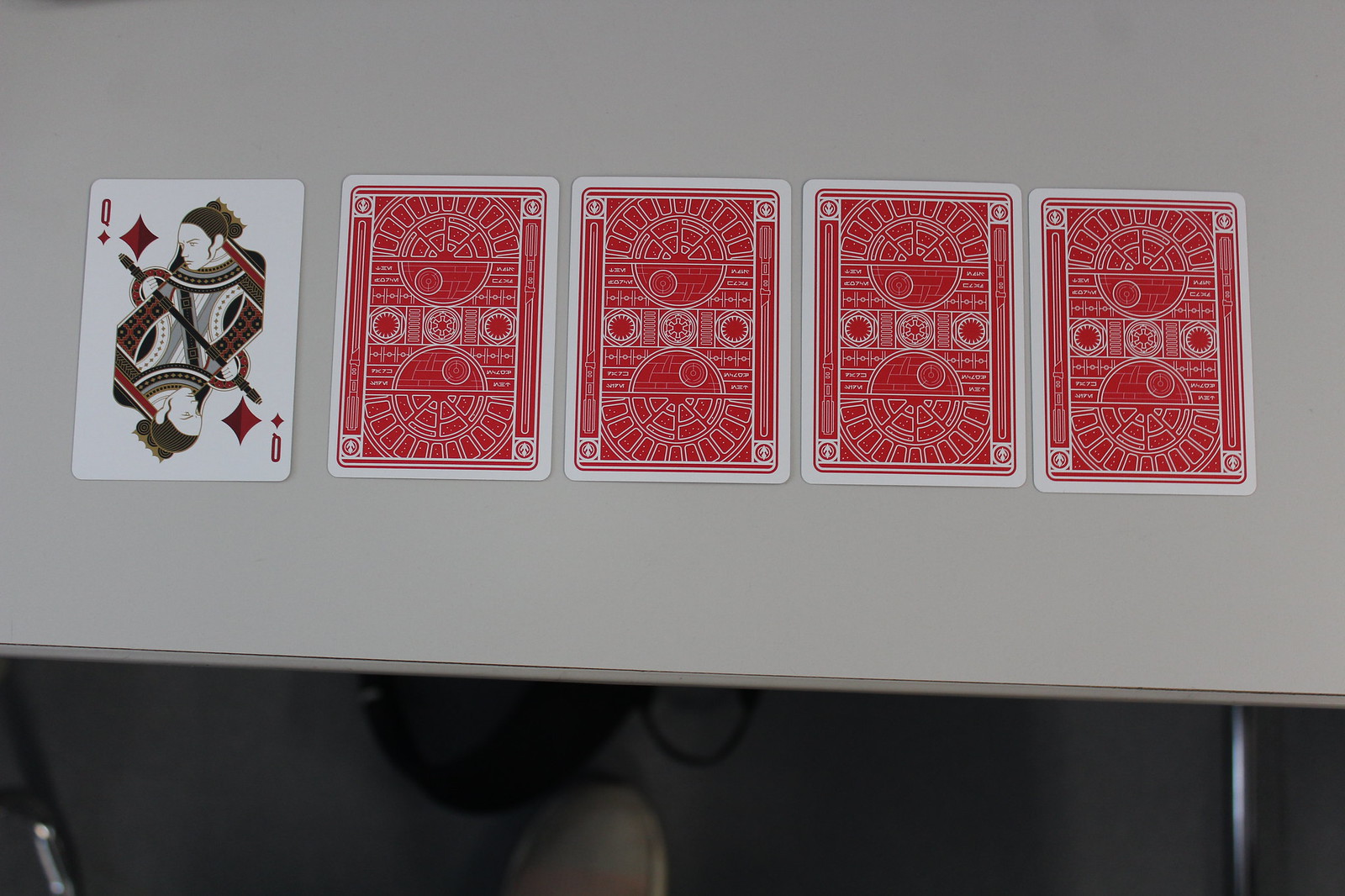This color photograph features five playing cards from a traditional deck. The backside of each card displays a red and white design that resembles intricate architectural patterns. Four of these cards are arranged neatly side by side, closely aligned in a precise row. To the left of this quartet, an additional card is set face up, revealing the Queen of Diamonds. This Queen is depicted in a classic style, mirrored to show her from both top and bottom perspectives, and adorned with ornate embellishments and the distinctive diamond symbol.

The arrangement of the cards is approximately four inches from the edge of a white laminate desktop. In the background, part of a metal support structure for the desk is visible. Additionally, the top of one shoe can be seen on the floor, hinting at the presence of the person seated at the desk and handling the cards.